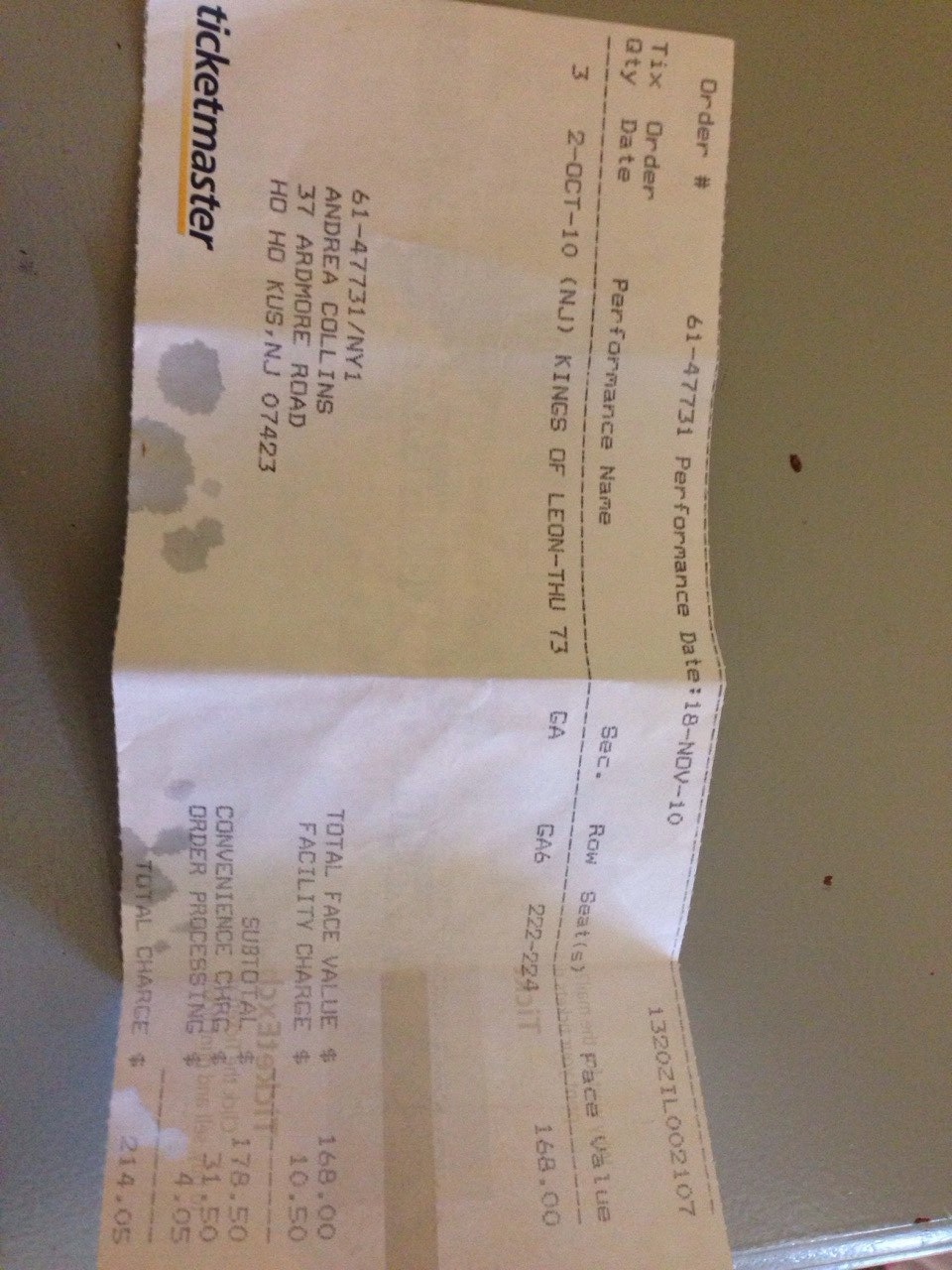This image depicts a Ticketmaster receipt addressed to Andrea Collins at 37 Ardmore Road, HoHo Coos, New Jersey, 07423. The receipt is laid out on a gray table and aligned vertically. It details the purchase of general admission tickets for the Kings of Leon concert on October 2, 2010. Specifically, the tickets are for Row 6, Seats 222-224, with a face value of $168. Additional charges include a facility fee of $10.50, a Ticketmaster fee of $31.50, and an extra charge of $4.05, bringing the total cost to $214.05. The Ticketmaster logo is prominently displayed at the bottom right corner of the receipt, highlighted by a yellow streak. The receipt appears to have several numbers and letters scattered across it, suggesting it was previously enclosed in an envelope for mailing.